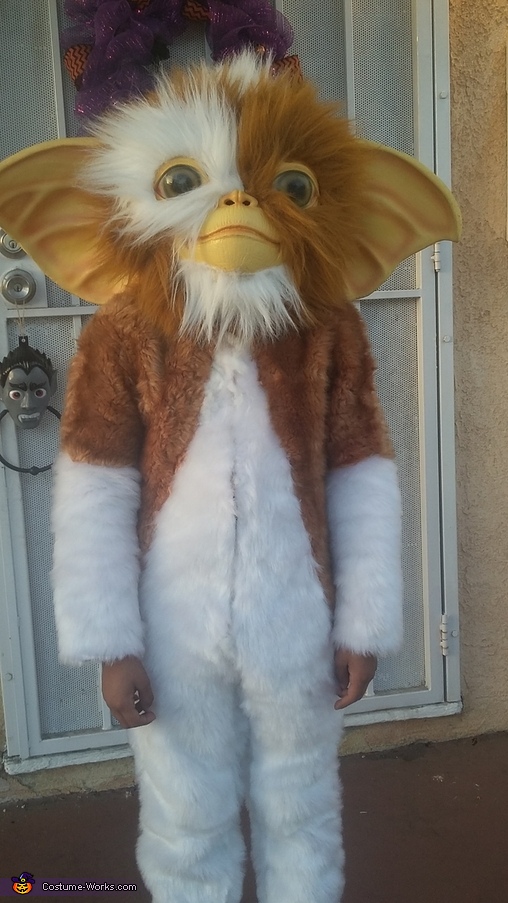In this vibrant Halloween image, taken outdoors during the daytime, a young boy stands in front of a white screen door adorned with a purple wreath and a vampire head decoration over the doorknob. He is dressed in an impressively detailed costume of Gizmo, the adorable character from the movie *Gremlins*. The costume features a furry bodysuit with brown shoulders extending down the sides to the waist, contrasting with white fur on the forearms, the center of the waist, and the legs, leaving the child's light brown hands visible. The headpiece of the costume is a full helmet modeled after Gizmo’s head, showcasing a mix of brown and white fur, large leaf-like ears, lifelike eyes, and a face with a white and brown split and a white scruff on the chin. This delightful scene is further enhanced by a small jack-o'-lantern emoji with a witch's hat in the lower left corner, accompanied by the website name “Costume-Works.com” written in white print with a black outline on a purple background, suggesting this image might be featured on a costume rental or showcase website.